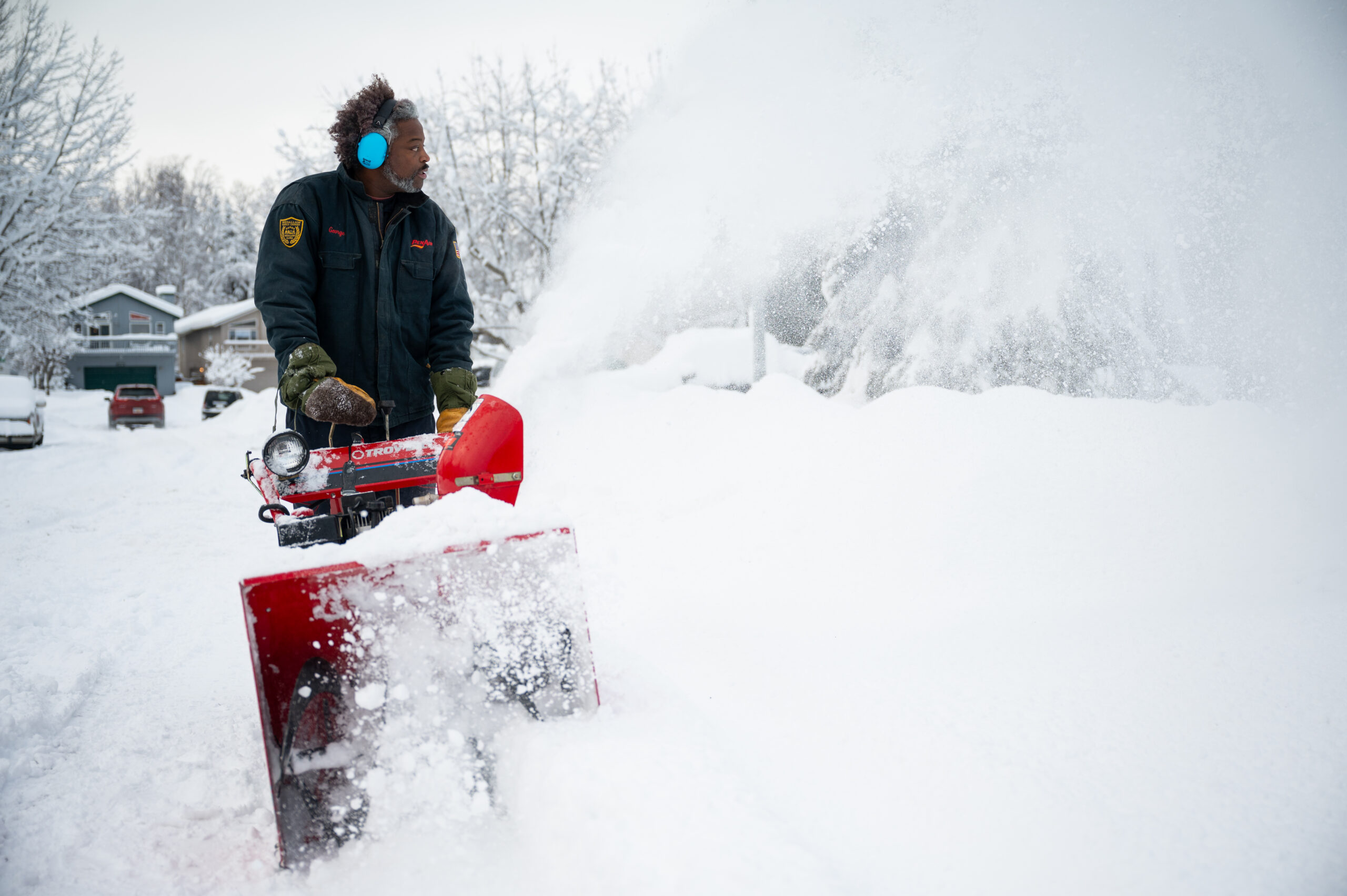In this landscape-oriented color photograph, an African-American man is depicted on the left side of the image operating a red snow blower on a snow-covered driveway or road. The man, who has long kinky black hair, a white beard, and is wearing blue earmuffs, heavy gloves, and a black and blue jacket, stands near the foreground with his hands on the machine. The snow blower features a horizontal piece at the top with a headlight and a chute opening that spews a stream of white powdery snow toward the upper right portion of the image. The background reveals a scenic winter landscape with snow-laden trees in the upper left, a white sky above, and a few two-story houses with snow-covered roofs and driveways, as well as cars including a gray and brown house and a red car partially buried under the snow. The scene captures the realism of a snowy day outdoors with the man diligently clearing the path amidst a picturesque, snow-blanketed environment.